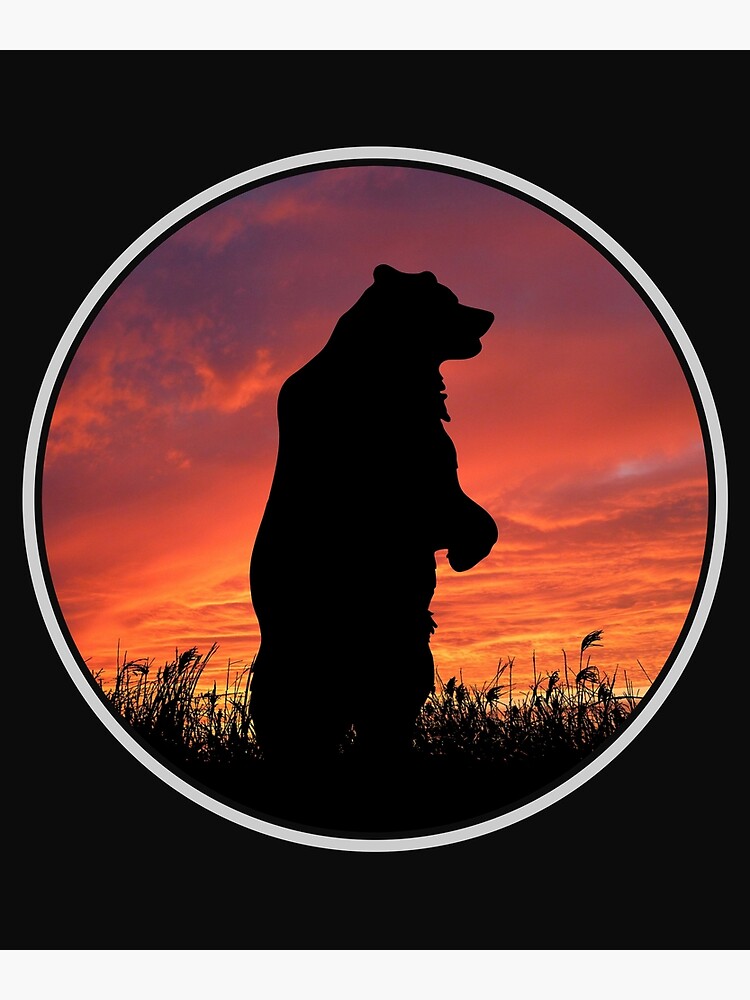The image showcases a detailed artwork of a bear standing on its hind legs, set within a circular central picture bordered by a thin white ring. The bear is depicted as a pure black silhouette, facing towards the right. The ground below it is also a silhouette adorned with black shrubbery and tall grasses. The background sky is filled with densely packed, thick clouds illuminated by the rich hues of an amber-yellow and reddish-orange, resembling a vibrant sunset. The overall rectangular image is dominated by a dark, black backdrop, highlighting the circular bear artwork at its center.